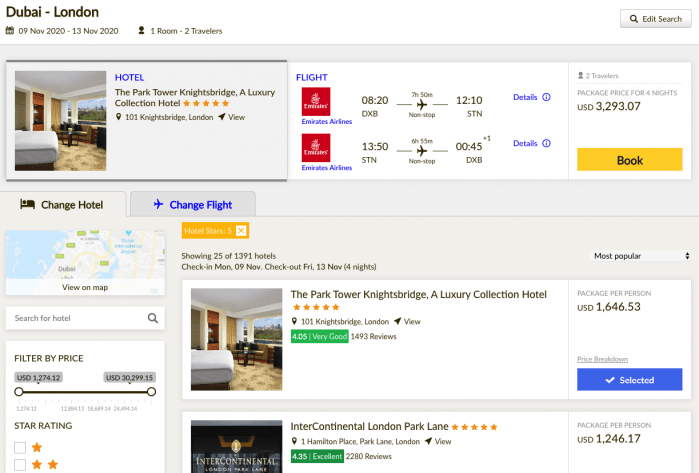The image appears to be a screenshot of a housing or rental website, possibly focused on both accommodation and flight bookings. The page showcases a search for accommodations in Dubai and London, specifying travel dates from September 9, 2020, to November 13, 2020. The active filter is set to one room for true travelers.

In the accommodation section, there is a listing for "The Park Tower, Knightsbridge, a Luxury Collection Hotel" which boasts a five-star rating and is located at 101 Knightsbridge, London. An option is provided to view the hotel details.

In the flight section, details for an Emirates Airlines flight are displayed. The departure time is 08:20, and the arrival time is 12:10. The cost of the flight is USD $3,293.07, with a clickable option for more details and a “Book” button.

At the bottom of the page, there are options to change the hotel or flight, view a map, and filter results by price and star rating. The user can filter by price using a sliding scale and select hotels based on star rating from one to five stars.

In the center, it shows a summary: displaying 25 of 1,391 hotels with check-in on Monday, November 9, and check-out on Friday, November 13, for a total of four nights. Two hotel options are prominently displayed: "The Park Tower, Knightsbridge, a Luxury Collection Hotel," priced at $1,646.53, and "Intercontinental London Park Lane," priced at $1,246.17.